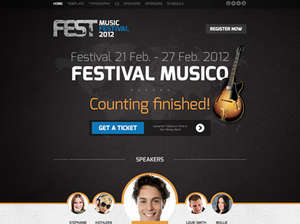This image is a promotional screenshot for the Fest! Music Festival 2012. In the upper left-hand corner, the text "Fest, Music Festival 2012" is prominently displayed. On the upper right-hand corner, there is a small, somewhat difficult-to-read button that says "Register Now." 

The main section of the image features the event dates, "Festival 21 February to 27 February 2012." Below, the text reads "Festival Musico," followed by "Counting Finished," indicating that a countdown presumably for the event has ended. To the right, there is an image of an electric guitar, adding a musical touch to the festive feel.

At the bottom, a noticeable blue button invites viewers to "Get a Ticket," beneath which there are five images of speakers in a lineup. The central figure is a person with lighter skin and black, fluffy hair. Flanking this person on the left are two light-skinned females, while on the right are a light-skinned male and another light-skinned female.

Overall, this image captures the promotional essence of the Fest! Music Festival 2012, complete with event details, ticket prompts, and visual highlights of musical elements and featured speakers. The countdown has concluded, reflecting its 2012 timeline.